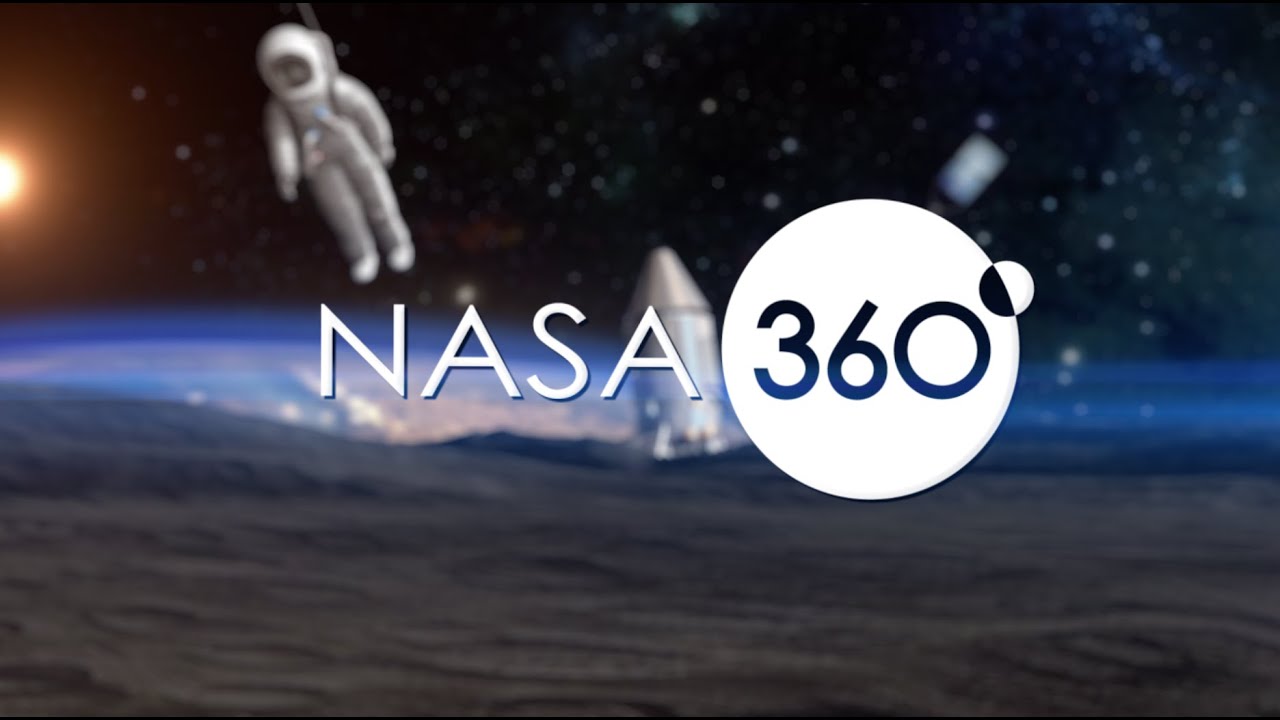The image shows a scene reminiscent of space exploration, likely a digital rendering, featuring various detailed elements. The bottom third of the image represents the surface of a planet that is not Earth, colored in shades of brown with a blue haze. The background shows a black night sky peppered with stars. At the very top left, there's a depiction of the Sun, partially cut off.

In the center of the image, prominently displayed, is the text "NASA 360". The word "NASA" is in thin, white, all-capital letters, while "360" is inside a white circle with the numbers appearing cut out, revealing the background image through them.

Positioned centrally behind the text and extending slightly to the right is a rocket ship or lunar lander. Additionally, more towards the top left of the image, there is a figure in a white space suit with a helmet, seemingly floating.

In the middle background, behind the alleged shuttle, appears to be Earth or another celestial body, contributing to the cosmic setting. The overall composition and stylistic elements suggest this image is used in an advertisement for NASA 360, a program related to space exploration.